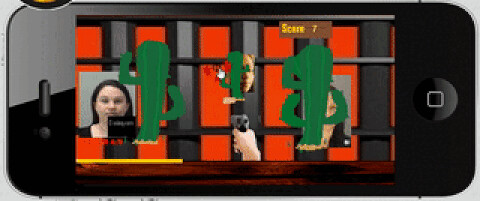This detailed caption has been cleaned up and formulated based on the given voice description:

"An illustration or screenshot from a video game displayed on a vintage Apple phone screen, characterized by a distinctive home button on the right-hand side. The phone's background is predominantly black, with a touch of medium gray in the upper left corner. The game itself features a vividly colored background comprising shades of orange, black, and gray, reminiscent of an office building's facade with orange windows contrasting against the structural black and gray elements. In the foreground, three portraits of faces are visible, each positioned behind a cactus. A hand holding a handgun is visibly aimed at the center cactus, with the gun discharging at the target."